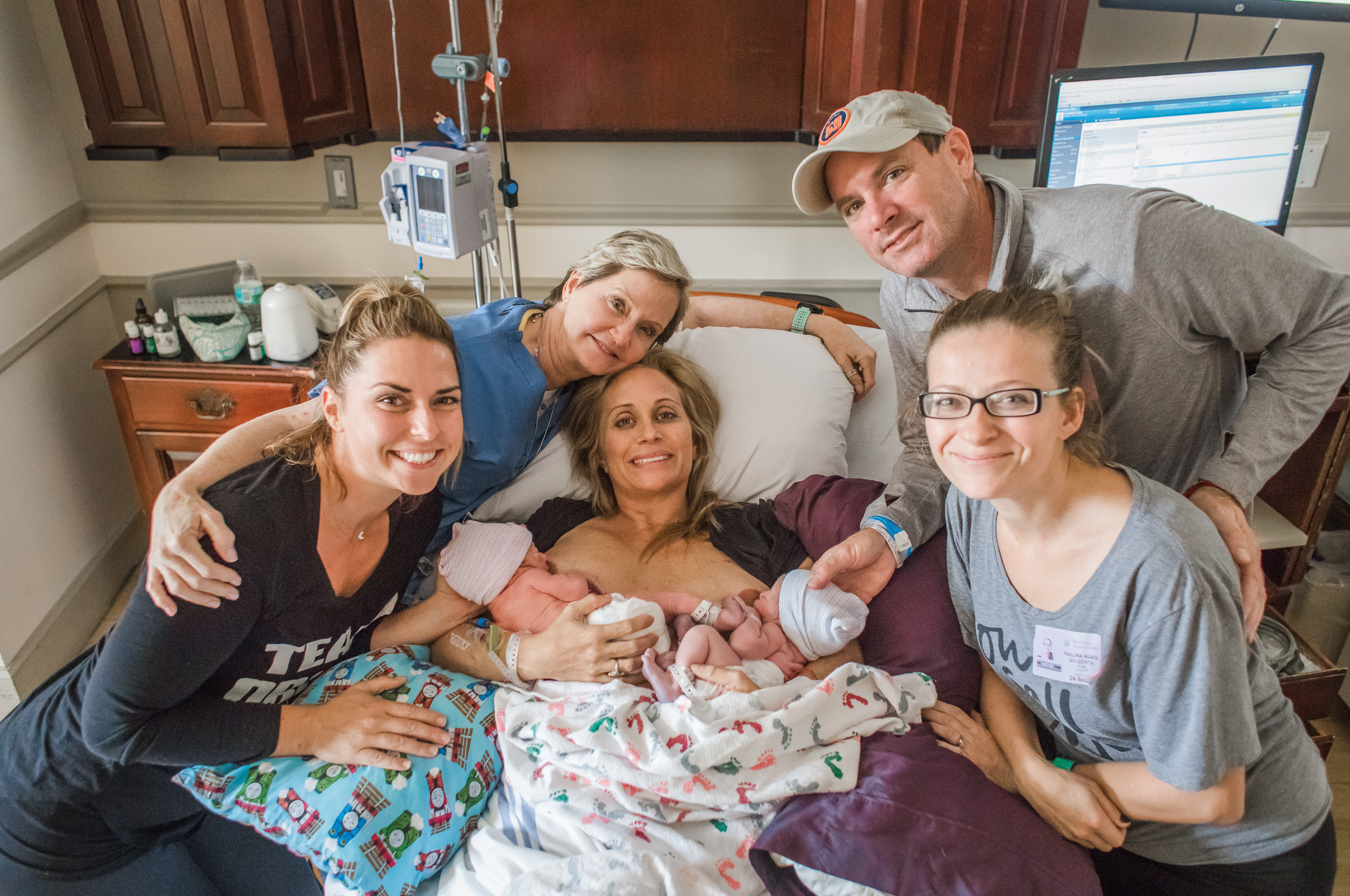In this heartwarming photograph, we witness a touching moment as a family gathers around a new mother who has just given birth to twins. The mother is lying in a hospital bed, attentively breastfeeding her newborns, who are cozily dressed in hats and diapers. Surrounding her are four family members—each radiating joy and support. 

To the right of the mother, a woman with glasses and her hair tied up, dressed in a gray t-shirt, stands closest. This woman appears to be caring and vigilant, possibly wearing some kind of identification badge. Behind her, a man donning a gray long-sleeved shirt and a hat tenderly places one hand on the mother and another on one of the babies. 

On the left side, another smiling woman in a black shirt looks directly at the camera, her expression full of happiness. Beside her, an older woman wearing a blue shirt embraces her warmly, symbolizing the closeness and support of family. The hospital setting is evident with brown cabinets lining the room, medical equipment, and a computer screen towards the right, along with personal items like oils placed on the nightstand, adding a touch of home to the clinical environment. This image beautifully encapsulates the joy and togetherness of family at the arrival of new life.